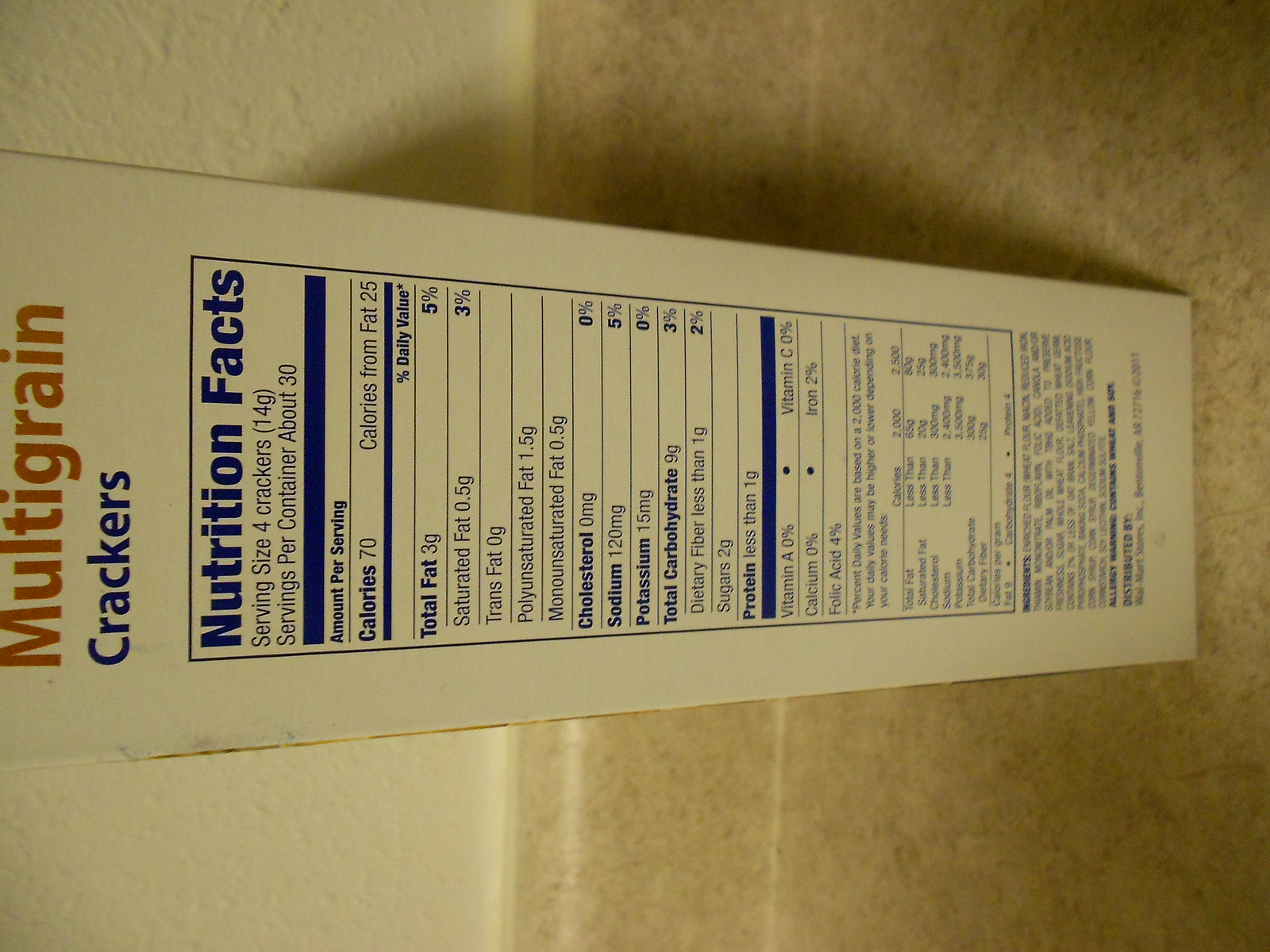In the image, a rectangular box of multi-grain crackers is positioned on its side atop a counter. The box's top is oriented to the left owing to the sideways flip of the image. The counter beneath the box displays a yellowish hue, complemented by a similarly colored yellow wall in the background. 

The box prominently features the text "Multi-Grain Crackers," with "Multi-Grain" highlighted in red and "Crackers" in blue. Other textual details on the box are presented in blue font. Some visible information includes the nutritional facts: a serving size of 4 crackers weighing 14 grams, approximately 30 servings per container, 70 calories per serving with 25 calories from fat. Additional nutritional details continue down to the bottom of the box, listing the ingredients in very small, barely legible print.